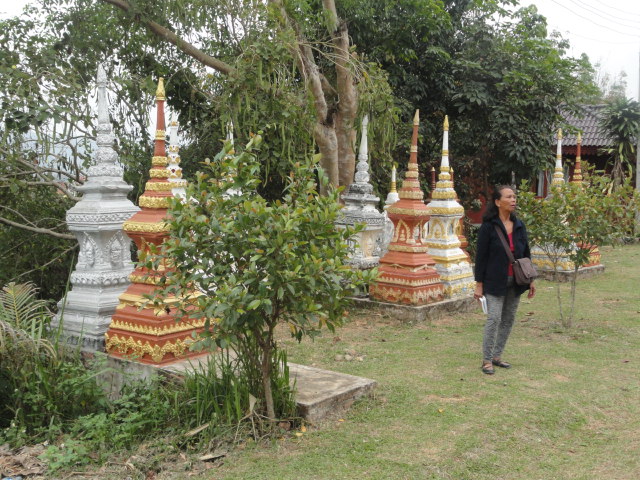This photograph captures an Asian Buddhist shrine featuring a series of small, ornate structures resembling miniature pagodas or temple towers. The towers start thick at the base and taper off as they rise, with some painted in plain cement white, others in vivid red and gold, and yet others adorned with white and gold trim. Positioned on concrete slabs, these structures stand out against the backdrop of a lush garden and tall trees, contributing to the serene, spiritual ambiance of the site.

On the right side of the photograph stands an Asian woman with black hair pulled back, dressed in a black jacket, gray pants, and black shoes. She also wears a red shirt beneath her jacket and carries a purse slung across her shoulders. The woman appears to be mid-speech, facing to the right, adding a human element to the tranquil scene. The ground she stands on is covered with well-mowed grass interspersed with patches of dirt, further highlighting the natural and maintained beauty of the religious complex that surrounds her.